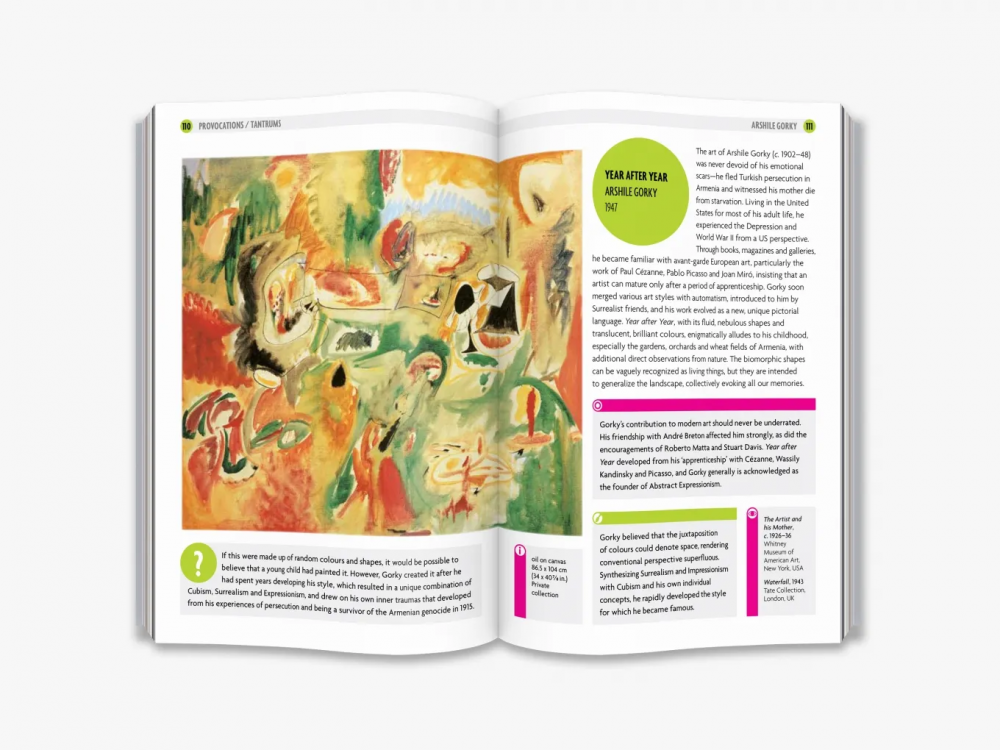The image depicts an opened book, revealing a two-page spread featuring an abstract painting titled "Year After Year" by Arshav Gorky, dated 1947. The artwork dominates the left page with a vibrant palette of greens, reds, blues, oranges, yellows, and blacks, blending to form an enigmatic scene that hints at a dinner or farm setting, though its abstract nature renders it open to interpretation. The right page contains text printed in dark blue ink on a white background, separated by a thick orange line. The text highlights Gorky's emotional and tumultuous life, including his escape from Turkish persecution in Armenia, his mother's death from starvation, and the impact of the Depression and World War II. It notes Gorky's influence from European avant-garde artists like Paul Cezanne, Picasso, and Jean Miró, and his development of a unique abstract style influenced by surrealist automatism. A small, round disc near the painting provides the name, artist, and year of the artwork. The overall layout and detailed context underscore Gorky's significant contribution to abstract art and his intrinsically emotional creations.